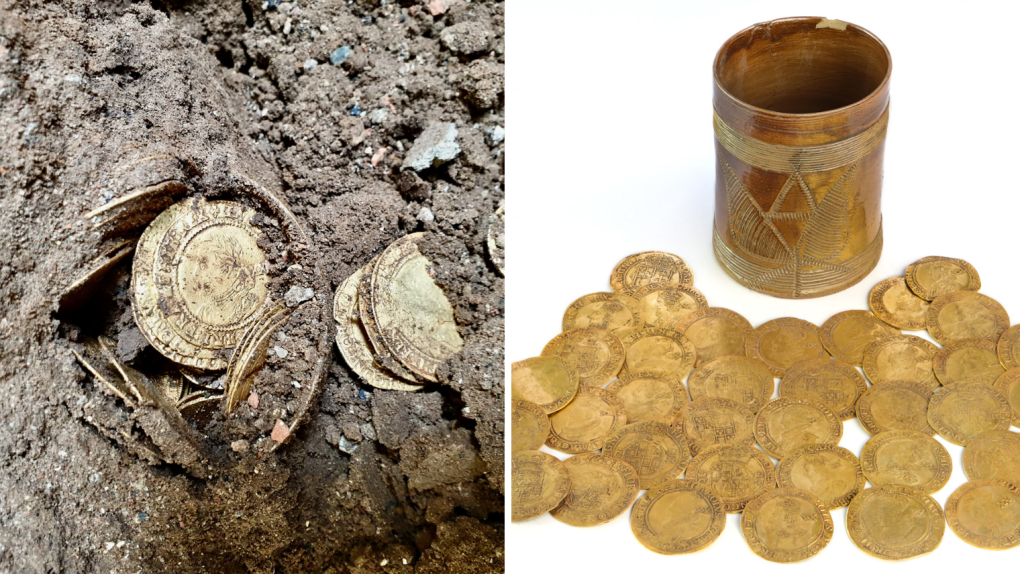The image features a pair of contrasting photographs depicting an apparent treasure discovery. On the left, a 'before' scene presents a cluster of gold coins partially buried in wet, muddy, dark brown soil, contained within a discernible container. The soil exhibits a wet, dark brown shade, giving a rich background to the glimmering, ancient-looking coins. These coins appear circular, thin, flat, and are marked with indistinct text or symbols.

On the right, the 'after' scene, set against a stark white background, showcases approximately 25 to 30 meticulously cleaned gold coins, now shining brightly with all traces of mud removed. Accompanying the coins is a round, golden container adorned with a couple of bands and featuring beige scratch marks, suggesting a shiny mocha appearance. This container, hollow in the middle, seems to have housed the coins initially, adding a sense of historical treasure to the imagery. Overall, the detailed textures and colors in both scenes highlight the transformation from the initial excavation to the prized display of the found objects.